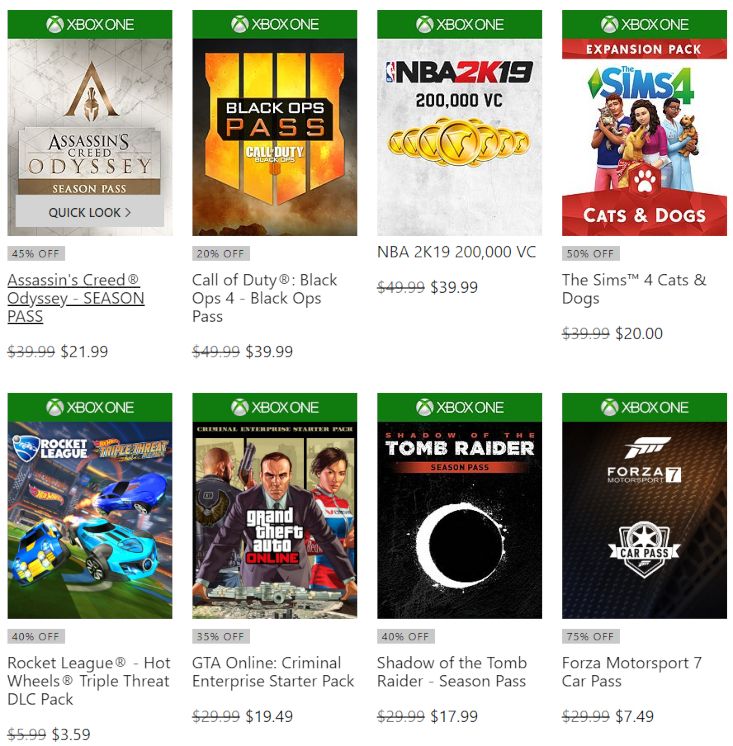Certainly! Here is a cleaned-up and detailed caption for the image:

---

The image displays two horizontal rows, each containing four Xbox game covers. Starting from the top left:

1. **Assassin's Creed Odyssey** - Includes a Season Pass. Originally priced at $39.99, it is now available for $21.99.
2. **Call of Duty: Black Ops 4** - Features the Black Ops Pass. The price has dropped from $49.99 to $39.99.
3. **NBA 2K19** - Offers 200,000 VC. Previously priced at $49.99, it is now $39.99.
4. **The Sims 4: Cats and Dogs Expansion Pack** - Originally $40.00, now on sale for $20.00.

In the bottom row, from left to right:

1. **Rocket League** - Hot Wheels Triple-Threat DLC Pack, discounted from $5.99 to $3.59.
2. **Grand Theft Auto Online** - Criminal Enterprise Starter Pack, with a reduced price from $30.00 to $19.49.
3. **Shadow of the Tomb Raider** - Season Pass, now $17.99, down from the original $29.99.
4. **Forza Motorsport 7** - Car Pass, significantly reduced from $29.99 to $7.49.

All game listings feature the green Xbox One cover and logo at the top of the game covers.

---